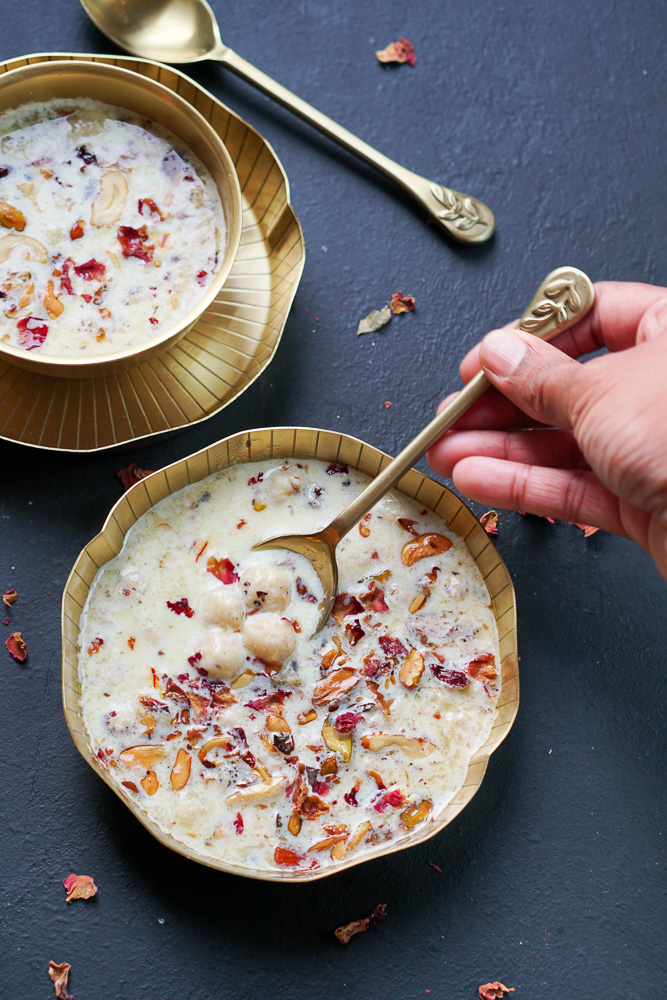The image shows a blue-painted table with two golden bowls containing the same creamy, milky substance. The larger bowl is positioned in the bottom right corner, and the smaller bowl is slightly above it to the left. Floating in the milky base are various colorful elements, including red, yellow, off-white, and brown pieces, possibly fruit or flower petals, and four larger dough-like nuggets. Scattered around the table are rose petals or leaves, adding a decorative touch. A right hand extends from the middle-right side of the image, gripping a golden spoon that is dipped into the larger bowl. The spoons in both bowls are golden, matching the bowls. The overall impression suggests a beautifully styled meal, possibly a floral-infused dessert or oatmeal-like dish.